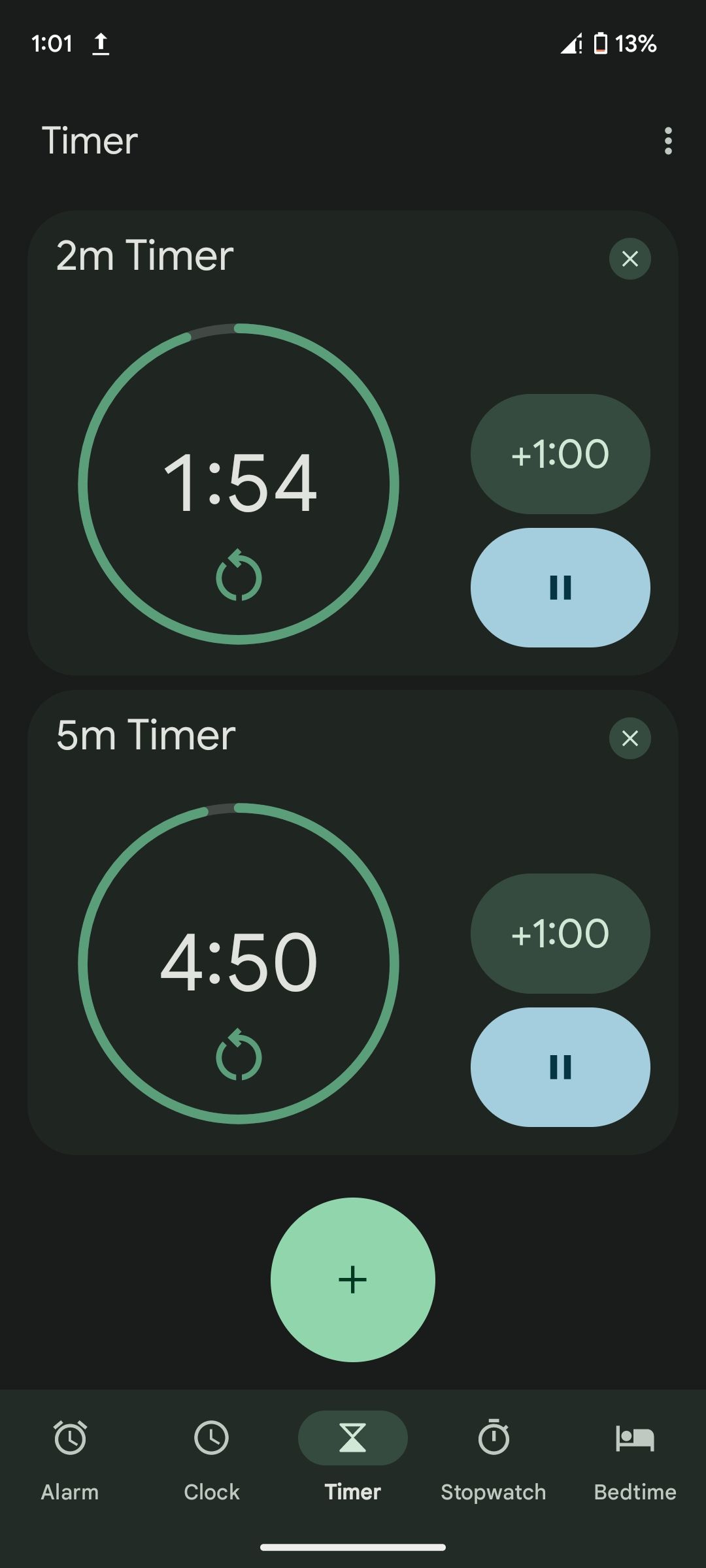A detailed screenshot of a smartphone's timer interface is shown. The top left corner displays '101' alongside an upload symbol, indicating the time or possibly an identifier. The phone has 3 out of 4 bars of data connectivity with a low battery of 13%. Just beneath this information, the screen shows a timer setup with a variety of features. 

A central green circle prominently displays '154' with a green refresh symbol, indicating an active timing session. Directly below this is a light blue pause button. Adjacent to it, a 5-minute timer is labeled with an 'X'. 

A second green circle on the right shows '450' with another green refresh symbol, and beside it, a gray circle encloses a '+1' sign with a teal pause button below. Another light green circle features a plus symbol, likely for adding more time. 

At the bottom of the interface, options for 'Alarm,' 'Clock,' 'Timer,' 'Stopwatch,' and 'Bedtime' are listed, with 'Timer' being highlighted. The rest of the screen features a stark black background, making the various components stand out sharply.